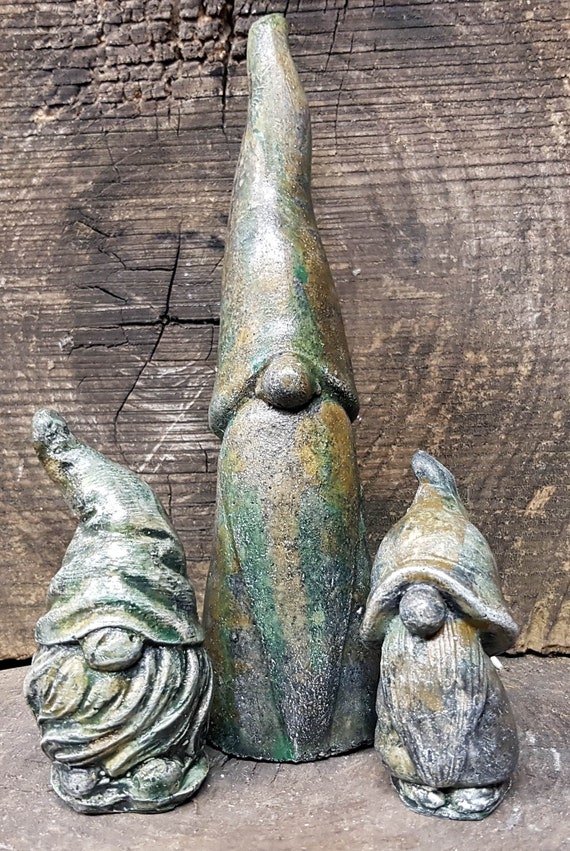The image showcases a detailed display of three gnome sculptures, carved from a material that gives them a patinaed, antiqued finish, possibly metal or wood. These gnomes are set against a backdrop of a large, cracked, and aged tree trunk, viewed axially, accentuating the rustic aesthetic. The three gnomes vary in height, with the middle one being the tallest and skinny. All of them sport tall, creased gnome hats that obstruct their eyes, leaving only their prominent noses visible. They have etched beards and wear garments that drape down to their feet. Their feet, some of which are shod in sandals, peek out from beneath their robes. The minimalistic yet intricate detailing of their features, including the beards and hats, reflects a blend of simplicity and craftsmanship.